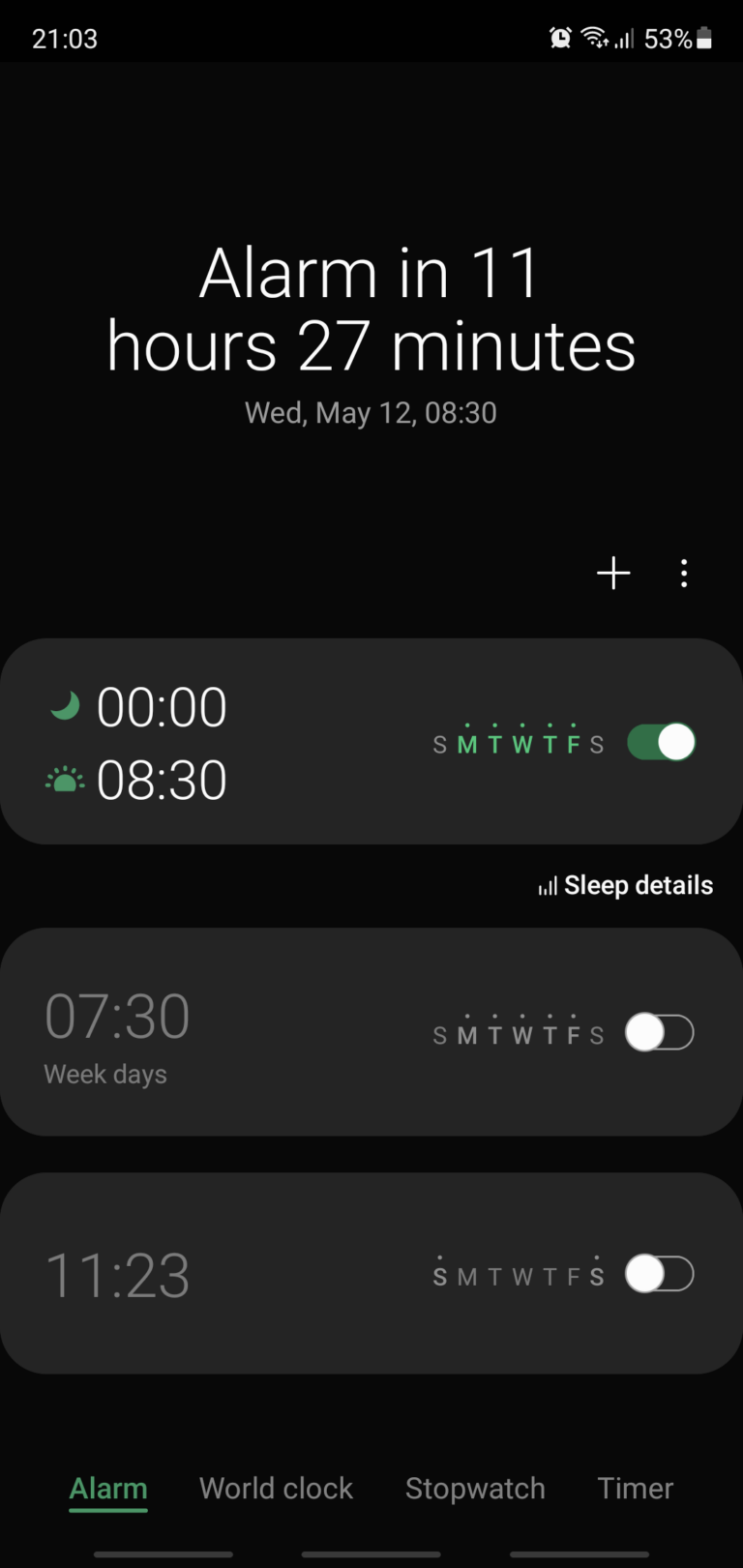The image is a screenshot of a smartphone's alarm interface. The screen is primarily black, with important elements displayed in white and green. At the very top, the status bar features the time "21:03" on the left and icons for an alarm, internet signal, and battery percentage (53%) on the right.

Centered below the status bar, large white text states, "Alarm in 11 hours 27 minutes," with a smaller, lighter font beneath it indicating, "Wed, May 12th, 08:30." There's a strip of black space, followed by a small white plus icon near the right, accompanied by three vertical dots.

The next section shows the current time as "00:00" with a small sun or moon icon in green next to it. Below that, a green sun icon precedes "08:30." Continuing down, there's a calendar row labeled "SMTWTFS," with Monday through Friday (MTWTF) in green and small green dots above them, while Saturday and Sunday (S and S) are gray. A green toggle switch on the right side indicates the associated alarm is active. 

Further down, white text reads "Sleep details," leading into another scheduling section, which displays an alarm set for "07:30 on weekdays." The corresponding calendar has gray letters and dots for Monday through Friday, and the toggle is switched off. Below this, an alarm set for "11:23" shows a similar calendar with dots over Saturday and Sunday, with its toggle also switched off.

At the very bottom of the screen, there is a menu with "Alarm" highlighted in green with an underline, followed by "World Clock," "Stopwatch," and "Timer," all in a light gray font.